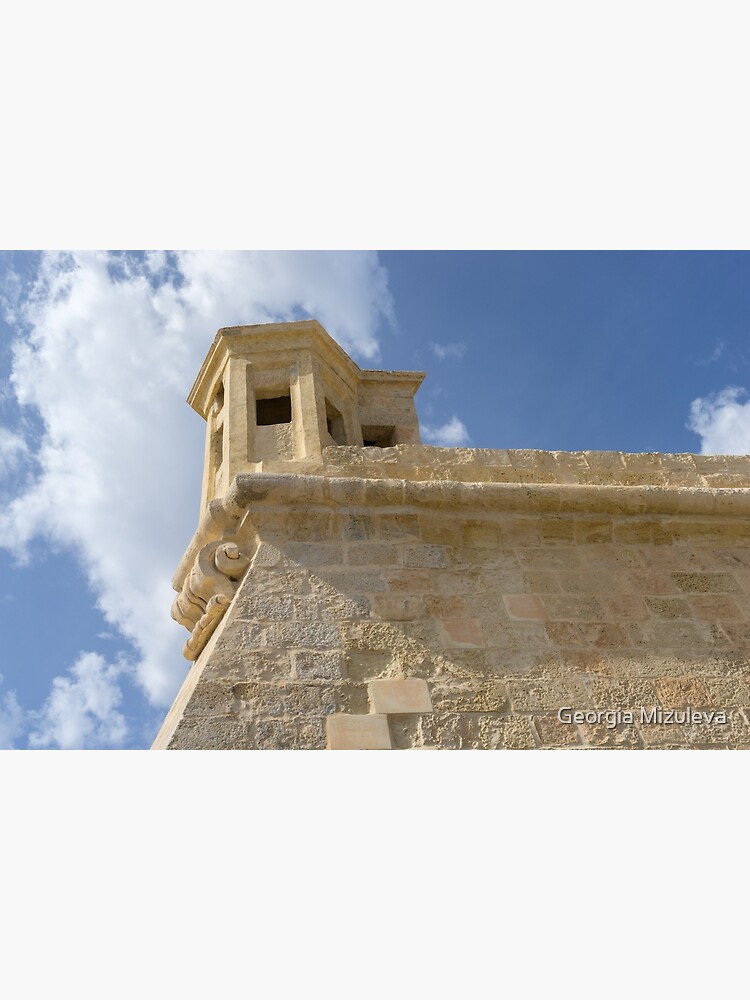This is a detailed side and upward view of an ancient, tan stone building with varied clay-colored bricks and stones. The structure is sandy brownish in color with some bluish and reddish hues. Starting from the bottom left, the building features a slanted front that rises slightly to the right, topped by a wave-like decorative stone protrusion. The side wall to the right has weathered, sandy brown bricks that lead up to a thin, canister-like brick detail wrapping around the structure. Above this, more brickwork continues, showing signs of erosion.

At the top, there is an ornate watchtower with a visible square window on the left and additional windows towards the front and right. This turret has a distinctive shape, almost octagonal, with square cutouts. The top stones jut out to form an edge, enhancing the antique feel of the building. Above the turret, a wall extends to the right, with a ledge protruding from its middle.

The sky forms a striking backdrop, predominantly blue with white cloud coverage to the left. Notably, the bottom right corner of the picture features the name "Georgia Misuliva."